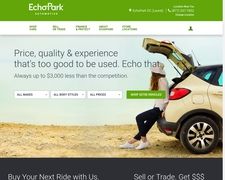The image depicts a screenshot set against a white background. At the top of the rectangular image is a thick green banner featuring light green text that reads "Echo Park." The remaining text to the right and below the banner is too blurred to be legible, but a telephone icon is vaguely recognizable. Below this, a white banner with green text is also present but equally illegible due to blurriness.

Centered in the screenshot is a color photograph of a woman interacting with the back hatchback of a tan vehicle that is oriented to face east. Only the rear portion of the vehicle is visible. The woman appears to be sitting with her butt inside the vehicle, wearing dark pants, white sneakers, a white long-sleeve shirt, and a white bucket hat. She has long dark hair, and her position reveals only the back of her head. Surrounding the photograph is additional text, some of which is discernible: "price, quality, and experience" and a promotional message stating, "Always up to $3,000 less than the competition."